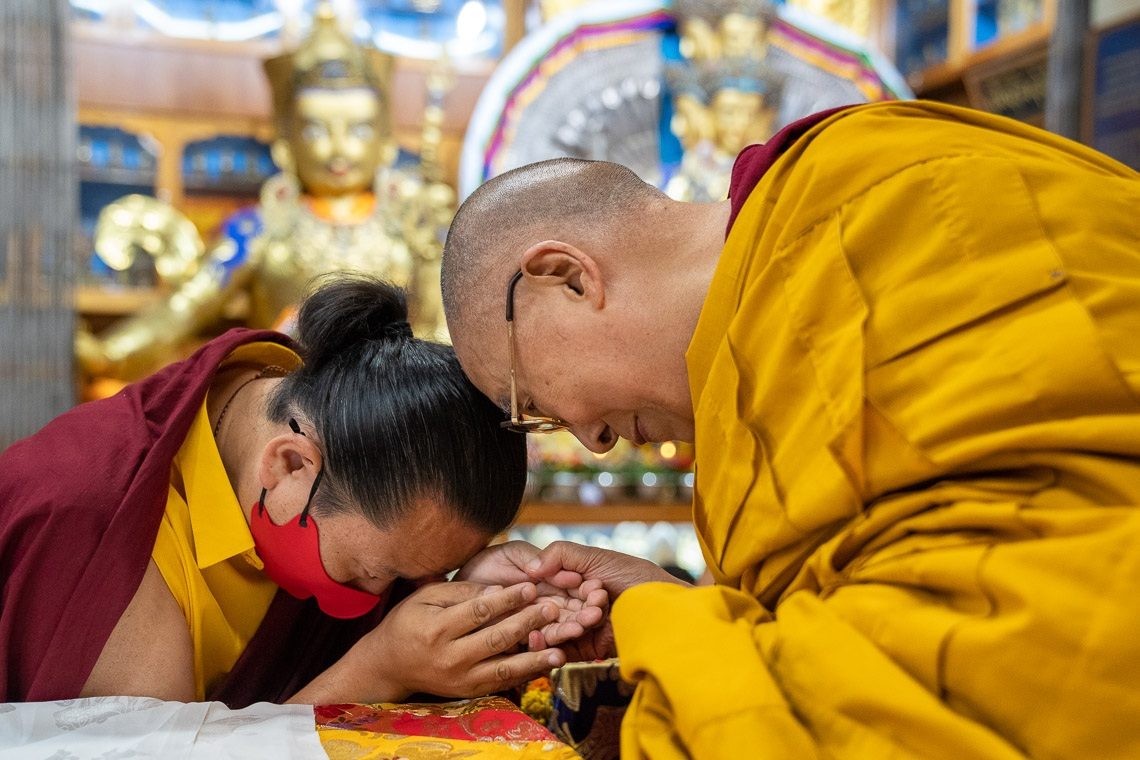In the heart of an ornate Buddhist temple, a touching moment unfolds between the Dalai Lama and another individual, possibly a fellow Buddhist monk. The Dalai Lama, distinguished by his gold-rimmed glasses and closely shaven head, wears a flowing mustard-yellow robe with hints of a crimson garment peeking out from the nape of his neck. He is bent forward, in a gesture of prayer, as he holds the hands of the other figure, characterized by long black hair tied in a ponytail. This person, dressed in an ochre shirt draped with a maroon cloth, bows his head in deep reverence, touching it to the Dalai Lama's.

The backdrop consists of opulent golden statues, notably a prominent Buddha figure adorned with a crown and jewels, surrounded by candles that enhance the sacred atmosphere. Though slightly blurred, the richly decorated walls and other colorful, possibly circular objects, add to the temple's grandeur. The scene is bathed in even lighting, highlighting the devotional interaction at the foreground, while the intricate and elaborate background remains slightly out of focus, underscoring the spiritual essence of the moment. A nearby table, covered with a white cloth and golden-brown decorative fabric, further enriches the setting of this sanctified space.